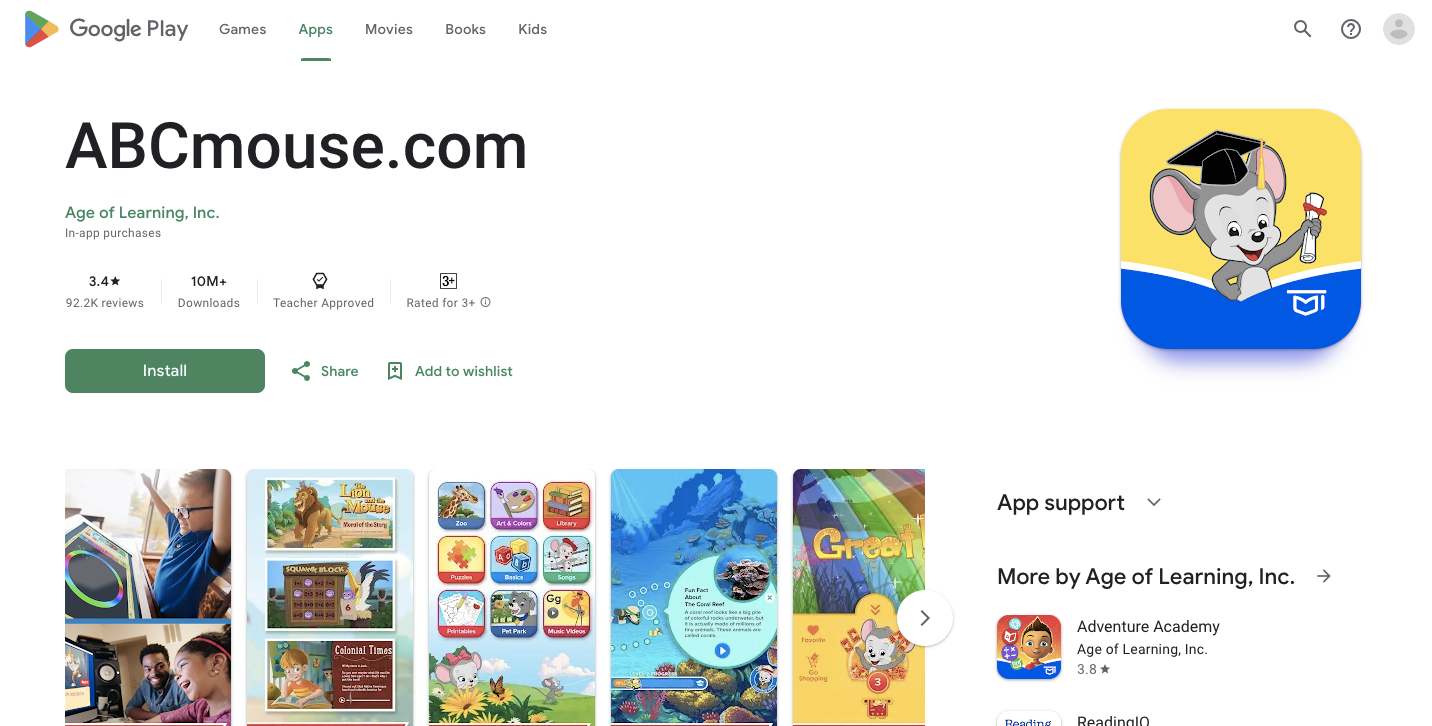This image captures a page from the Google Play Store, specifically highlighting the "Apps" section. Featured prominently is the app "ABCmouse.com" by Age of Learning, Inc., which offers in-app purchases. To the right of the app title, there is a small panel displaying a charming illustration of a grey mouse, characterized by pink inner ears, wearing a mortarboard, and holding a diploma, symbolizing education. Below this, there are several images showing children engaging with computers, accompanied by various thumbnails of animals and other visually appealing elements designed for young children. On the right side of the screen, there is an "App Support" button, followed by a section titled "More by Age of Learning, Inc." This section showcases other apps from the developer, including "Adventure Academy" which is rated 3.8 stars, and a partial thumbnail for "ReadingIQ."